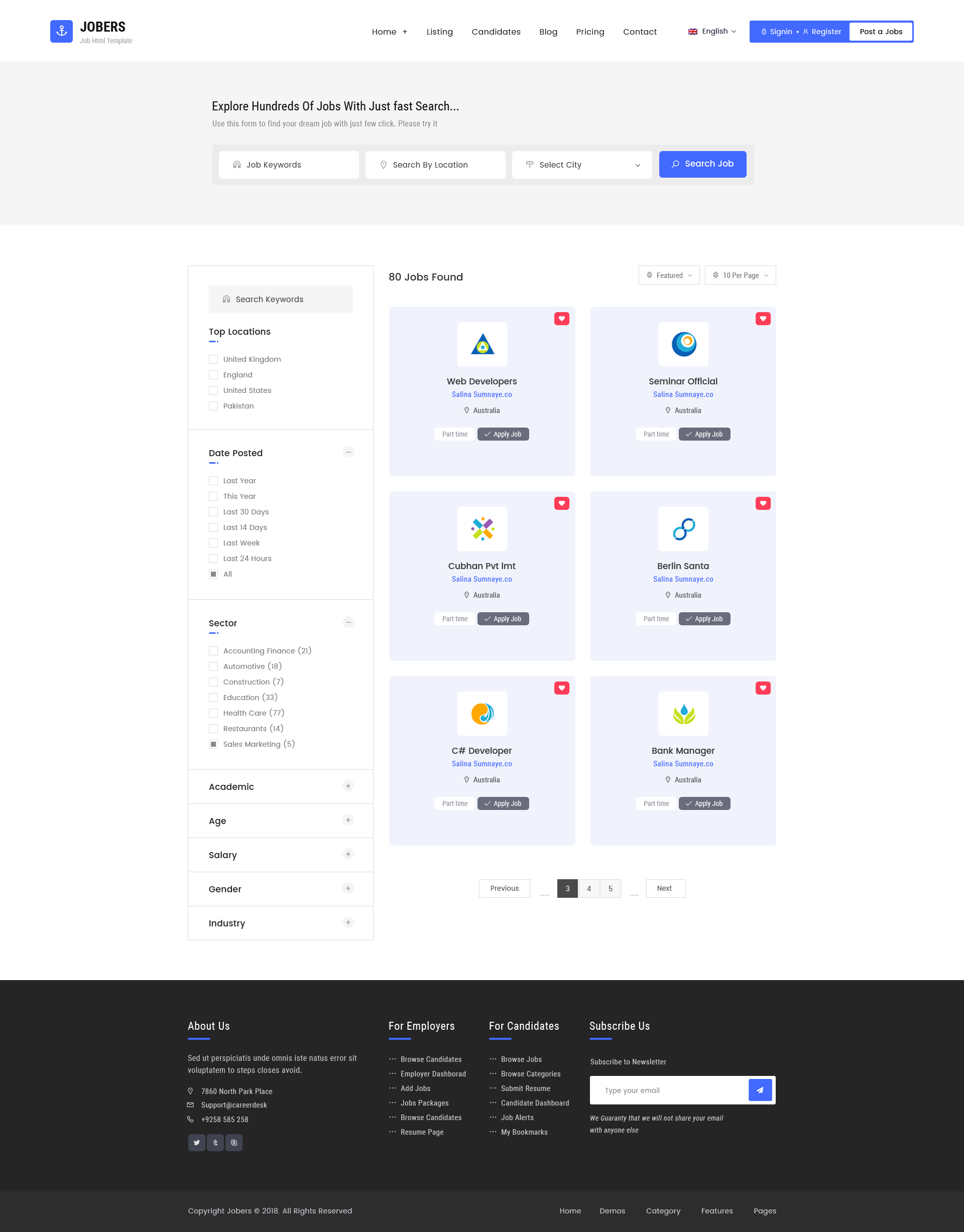The image features a white and light blue background. At the top, there is a white box with a small blue box inside, containing the text "Jobbers" next to it. The top section also includes several headings and a tiny red box. Below that, there are two buttons, one blue and one white.

In the middle, there is a prominent blue box with the text "Explore hundreds of jobs with just a fast search." Below this text, there are four buttons, three of which are white, and the last one is blue.

On the left side of the image, there is a white background with light blue outlines around the boxes. There are three smaller boxes, each accompanied by several headings and small down arrows. There is also a note indicating "30 jobs shared."

Below the note, there are two buttons followed by six blue boxes. 

1. The first blue box features a small green triangle, a pink box in the upper right corner with a white arrow, and two buttons at the bottom (one white and one blue).
2. The second box displays a globe icon inside a white box, the same pink box with the arrow, and two buttons at the bottom.
3. The third box contains a small yellow, blue, and purple flower, again with the pink box and two buttons at the bottom.
4. The fourth box has an '8' in blue within a white box, along with the pink box and arrow and two buttons.
5. The fifth box shows a yellow and blue circle and includes the pink box with a white arrow and two buttons.
6. The sixth and final blue box displays another yellow and blue flower, a pink box, and the standard two buttons at the bottom.

At the bottom of the image, there are numbers and a small button, ending with a large black square and what appears to be a search button.